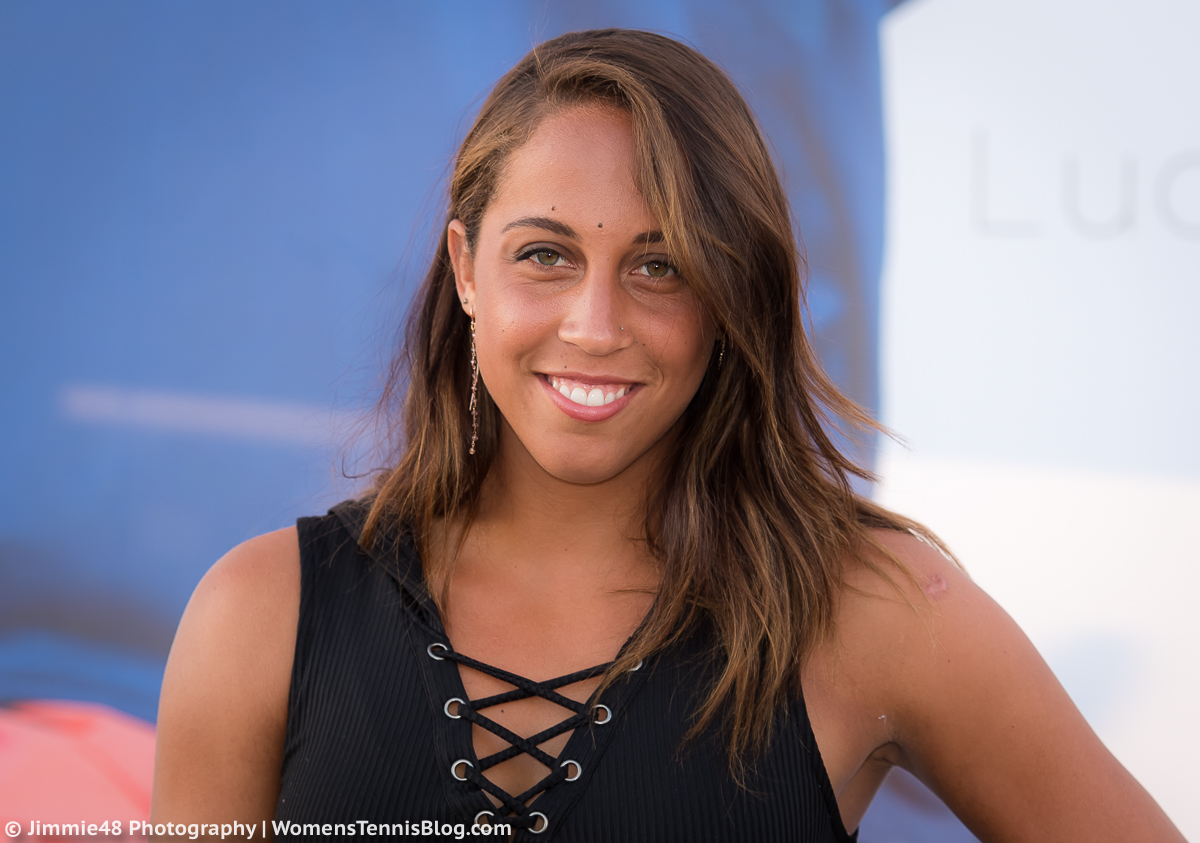A close-up photograph captures a confident Caucasian woman with a tan complexion and slightly wavy brown hair looking directly at the camera. She is wearing a black, textured tank top with a plunging V-neck, adorned with a lace-up crisscross pattern created by silver eyelet hooks down the front. Her earrings appear to be long, bead-like and possibly gold. The woman has notable large, white front teeth and is smiling, showcasing her light pink lipstick. Freckles are visible around and between her eyebrows. The background is blurred, featuring colors including white and light blue, suggesting it was taken outdoors with natural lighting. At the bottom left of the image, there is a white watermark reading "Jimmy 48 Photography, womanstennisblog.com."